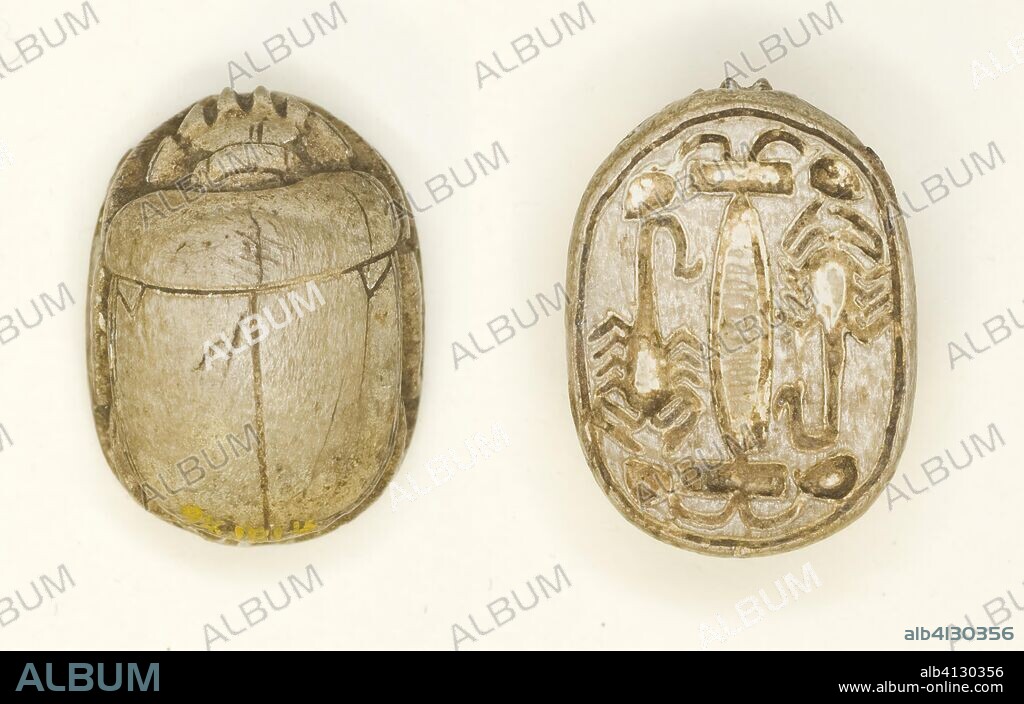The image features a detailed stock photograph of an ancient Egyptian scarab artifact, showcased from two perspectives—presumably the top and bottom of the same object. The upper view reveals a classic depiction of a scarab beetle with a distinct head, shoulders, segmented wings, and a central line down its back. The scarab is a shimmering gold or gold-like color, meticulously carved to emphasize its beetle-like features. 

In contrast, the bottom view is elaborately etched with fantastical images, including what appears to be a praying mantis and figures with numerous limbs, possibly scorpions or multi-armed human forms, stretching towards the edges. These intricate carvings are also rendered in the same gold or gold-tinted material, giving the entire piece an ancient and ornate look.

The artifact lies against a plain white or light tan background, which is watermarked diagonally with the word "ALBEM" to prevent unauthorized use of the image. Additionally, a subtle black rectangle at the bottom of the image contains the watermark "ALBEM" in light gray letters and includes a link to a website on the lower right corner. This photograph not only captures the artistic and historical essence of the scarab but also ensures the image's copyright protection through clear watermarks.